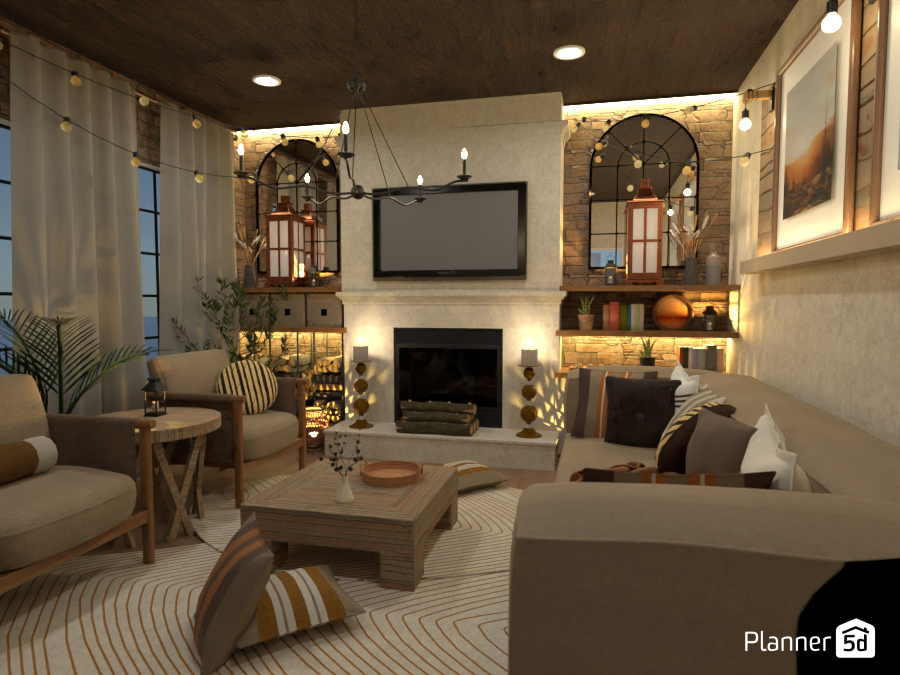The image presents a digitally-rendered living room scene, identified by the text "Planner 5D" in white within a small house icon in the bottom right corner. Dominated by a neutral color palette, the room features a high brown ceiling with recessed lighting. Two large windows with thick, long white drapes adorn the left wall, in front of which stand two tan chairs with wooden frames and grey cushions, flanking a small wooden table with a miner-style open lamp.

At the far wall, a prominent white fireplace serves as the focal point, with a large TV mounted above its mantel. On either side of the fireplace are brown sections of the wall, adorned with shelves and lighting beneath them, and rounded mirrors perched at the top. Flanking the fireplace are two lamps, and a few logs rest in front of the hearth.

Central to the room is a small brown wooden coffee table, set upon a white rug with a square golden pattern. Facing the two chairs on the left, a large grey couch with numerous colorful pillows fills the right side of the room. A painting hangs above the couch, and another painting is partly visible, cut out of the frame. The walls are cream or white colored, complementing the overall warm and inviting atmosphere of the room.